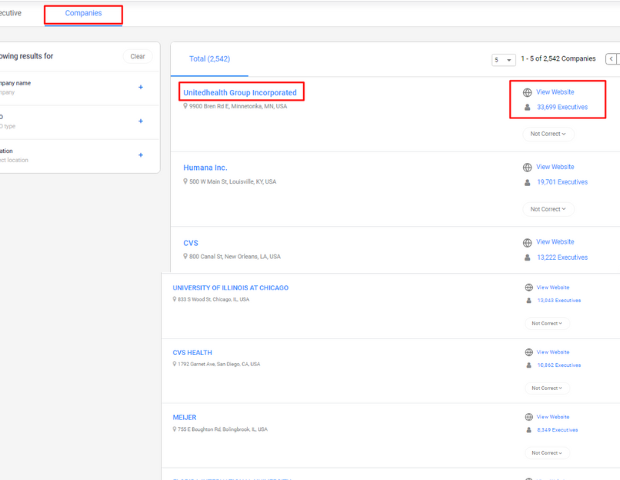The website features a straightforward design with a predominantly gray background and a slender, white tab running horizontally across the top of the page. The tab spans the entire width from left to right, containing blue text with the words "Companies," while the left side seems to be partially cut off but appears to say "Executive."

Below this tab, there is a smaller white box with the phrase "Showing results for" and a clear button to its right. Within this box, the company name is abbreviated, only displaying the letter "P" followed by a blue plus sign. Below it are two more truncated categories, each marked with a blue plus sign, one of which seems to pertain to location.

On the right side of this secondary box, the total number of results is displayed, which is 2,542. The companies listed below include detailed information for each entry:

1. **United Health Group Incorporated**
   - Location: 9900 Road East, Minnesota
   - Options: View Website, Executives (enclosed in a red box), and Not Connect with a dropdown menu.

2. **Humana Incorporated**
   - Options: View Website, Executives, and Not Connect.

3. **CVS**
   - Options: View Website, Executives, and Not Connect.
   
4. **University of Illinois Chicago**
   - Options: View Website, Executives, and Not Connect.

5. **CVS in San Diego**
   - Options: View Website, Executives, and Not Connect.

6. **Majar in Bolingbrook, Illinois**
   - Options: View Website, Executives, and Not Connect.

Each company listing includes 'View Website' and 'Executives' options, with the executives' count and a 'Not Connect' button encapsulated in red boxes. The section of the page displaying these company results has a white background, contrasting with the gray backdrop used across the rest of the site.